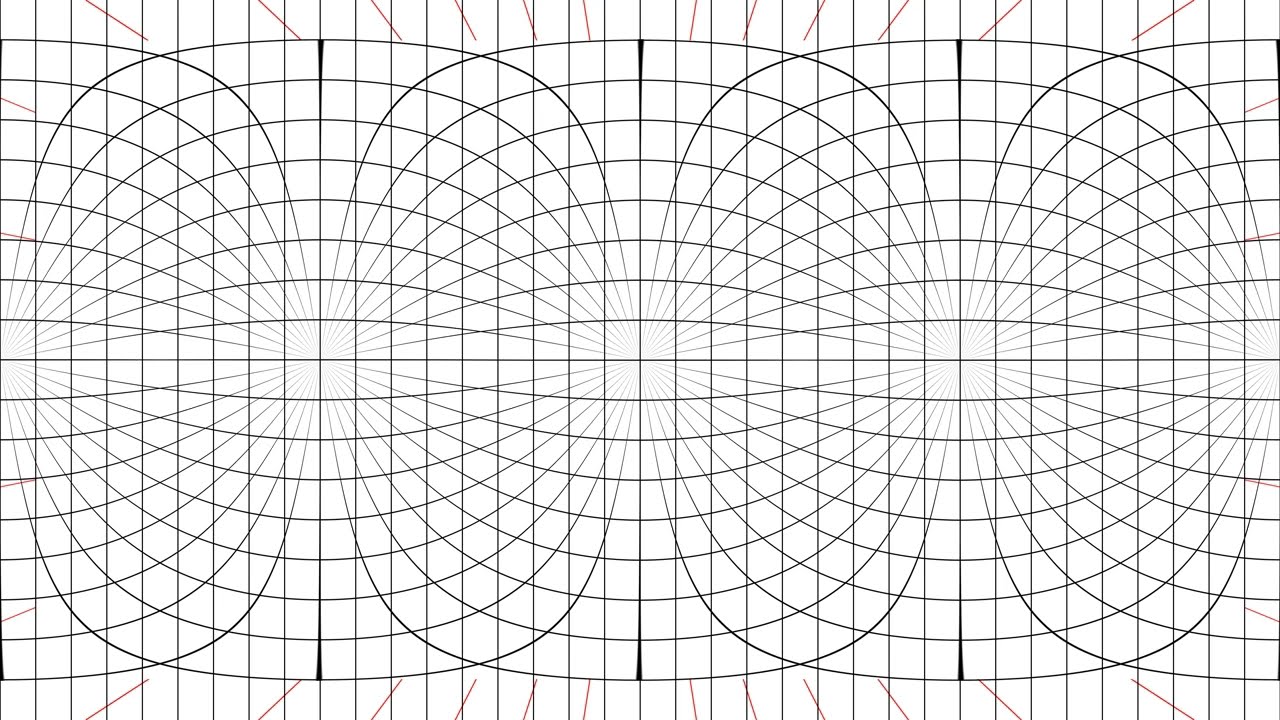The image is a computer-generated drawing featuring a detailed and intricate geometric pattern on a background resembling white graph paper. The grid consists of tiny squares created by horizontal and vertical black lines. Over this grid, a complex arrangement of overlapping large rounded squares and ovals is drawn. These shapes curve elegantly, forming a curvy look across the top of the image, each converging at central points from which lines radiate outward. The overall effect is a combination of three or four overlapping circles and three rounded squares, creating an elaborate network of curves and diagonal brown lines that contrast sharply with the black ones, enhancing the visual complexity.